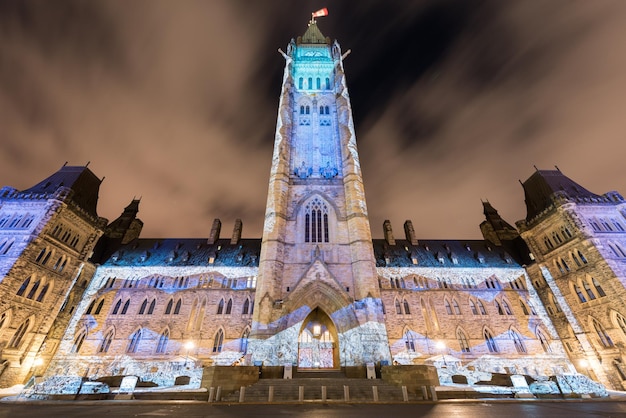This is an upward-looking photo captured from the base of an imposing, historical building that almost resembles a grand European palace or old castle. The image, taken at a steep angle under a dark, cloud-filled sky, shows the building symmetrically stretching across the frame, with its central tower soaring upwards. The tower, which appears to be about seven stories high, features a clock and is crowned with the Canadian flag—distinguishable by its two red stripes and central white stripe bearing a distant maple leaf. The building's exterior, likely gothic in style, is illuminated by a striking display of blue, brown, and white lights, giving it a festive or Christmas-themed ambiance. Additional architectural features include multiple arched windows consistent in design, with larger windows on the lower floors and smaller ones as you move higher up. Flanking the main tower are smaller towers, adding to the structure's grandeur. The combination of the building's detailed architecture and the dramatic lighting creates a stunning visual effect against the night sky.